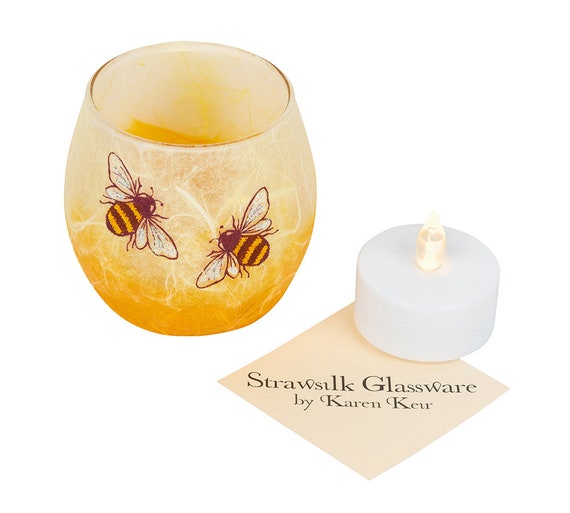The image features a vibrant candle holder and a battery-operated candle, set against a white background. On the left, a petite, round candle holder showcases an ombre design that transitions from lighter yellow at the top to a deeper orange at the base. Two detailed honeybees face each other on the surface of the candle holder, adding a charming touch. To the right, a thick, disc-shaped, battery-operated candle sits atop a square napkin positioned diagonally. The candle has a white base and a glass-like flame protruding from the center. The cream-colored napkin bears the inscription "Straw Silk Glassware by Karen Kure" in a fancy font.